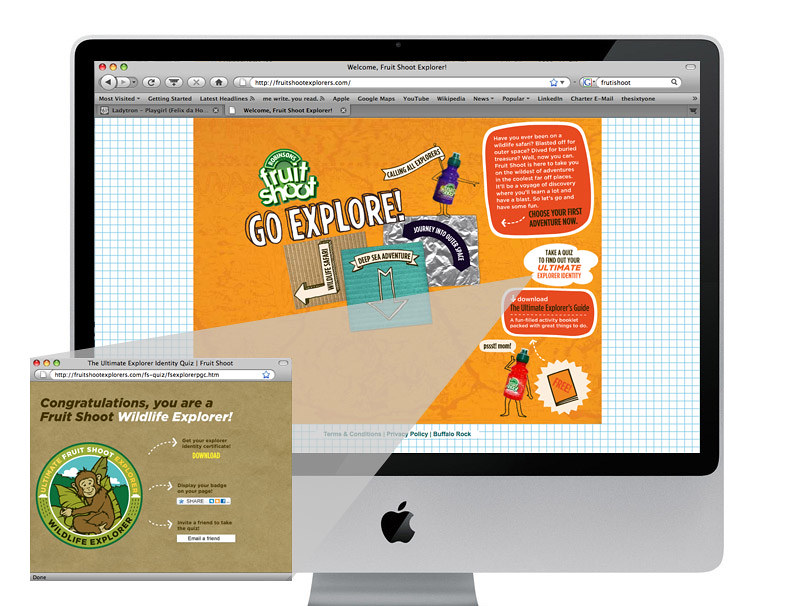The image is a detailed color photograph in landscape orientation, depicting an Apple computer monitor with a light gray bezel, featuring the Apple logo at the bottom center. On the screen of the monitor, a graphic design is visible, showcasing a web page for 'Fruit Shoot Go Explore.' The main section of the web page is dominated by an orange background with various colorful signs and text. Prominently at the top left, the 'FRUIT SHOOT' logo is displayed in green and white, while below it, the text 'GO EXPLORE!' is highlighted in white all-caps. Scattered across the page are icons including little bottles in purple and orange, and several text bubbles with unreadable content, suggesting a playful, kid-friendly interface.

In front of the monitor, a popup window is enlarged, bringing attention to an achievement message that reads, 'Congratulations, you are a Fruit Shoot Wildlife Explorer,' accompanied by a circular badge image featuring a monkey on a tan background. This badge has arrows indicating options to download, share, and promote it. The overall style presents a blend of photographic realism with graphical elements, merging a video-screenshot aesthetic with representational details.